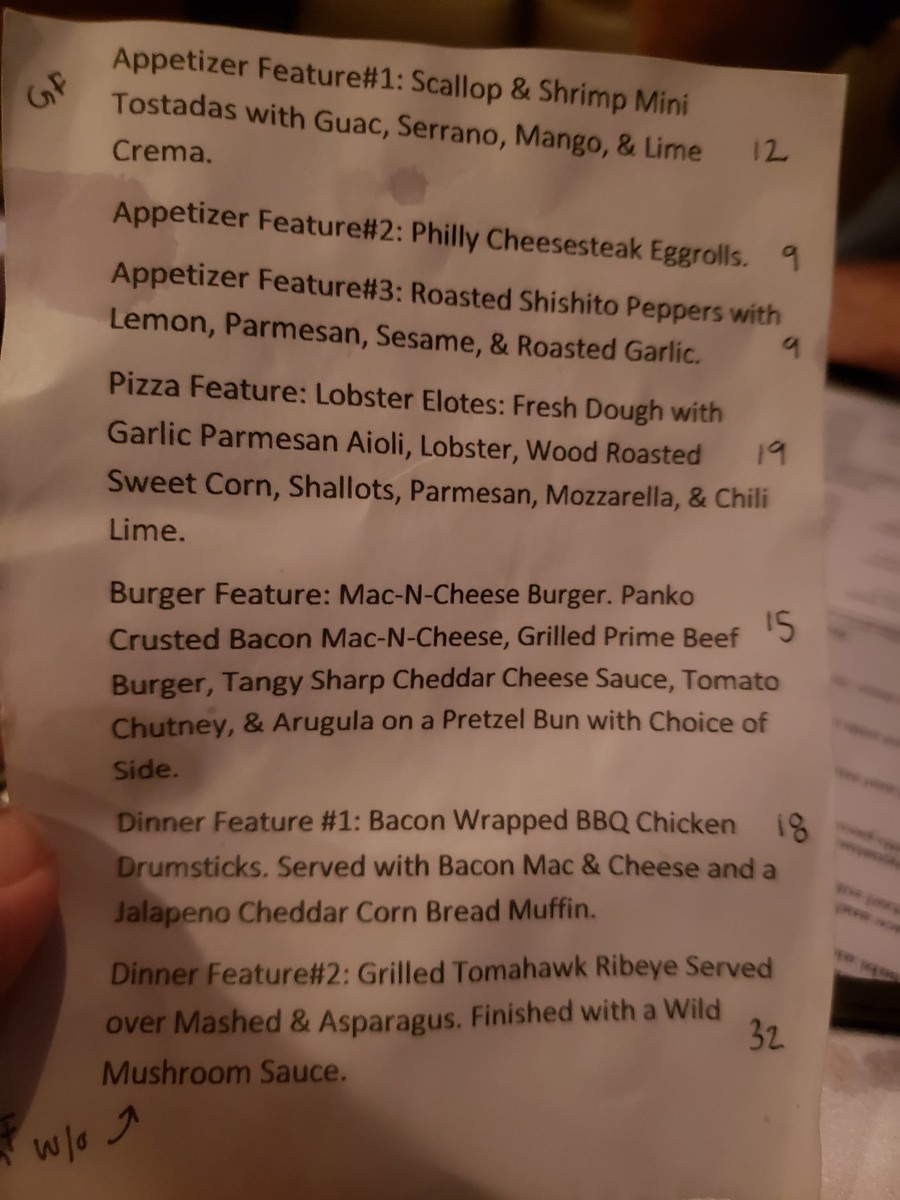### Café/Restaurant Menu Descriptions

#### Appetizers:
1. **Appetizer Feature #1** *(GF)*: 
   - **Scallop and Shrimp Mini Tostadas**
   - Ingredients: Guacamole, Serrano, Mango, Lime Crema
   - **Price**: 12 (currency unspecified)
   
2. **Appetizer Feature #2**:
   - **Philly Cheesesteak Egg Rolls**
   - **Price**: 9
   
3. **Appetizer Feature #3**:
   - **Roasted Shishito Peppers**
   - Ingredients: Lemon, Parmesan, Sesame, Roasted Garlic
   - **Price**: 9

#### Pizza:
- **Pizza Feature**:
  - **Lobster Elote**
  - Ingredients: Fresh Dough, Garlic, Parmesan Aioli, Lobster, Roasted Sweetcorn, Shallots, Parmesan, Mozzarella, Chili Lime
  - **Price**: 19

#### Burgers:
- **Burger Feature**:
  - **Mac and Cheese Burger**
  - Ingredients: Panko-Crusted Bacon Mac and Cheese, Grilled Prime Beef Burger, Tangy Sharp Cheddar Cheese Sauce, Tomato Chutney, Arugula, Pretzel Bun
  - **Includes**: Choice of Side
  - **Price**: 15

#### Dinner:
1. **Dinner Feature #1**:
   - **Bacon-Wrapped Barbecue Chicken Drumsticks**
   - Served with: Bacon Mac and Cheese, Jalapeno Cheddar Cornbread Muffin
   - **Price**: 18
   
2. **Dinner Feature #2**:
   - **Grilled Tomahawk Ribeye**
   - Served Over: Mash and Asparagus
   - Finished With: Wild Mushroom Sauce
   - **Price**: 32

#### Additional Note:
- Handwritten: "W/0 ↑" pointing to the mushroom in "Wild Mushroom Sauce" (context for "W" not provided).

### Important Notes: 
- The "GF" indicates Gluten-Free options.
- Prices are listed without specifying the currency.
- Handwritten note may require clarification from the establishment.

This detailed breakdown enhances comprehension and helps diners make informed decisions.